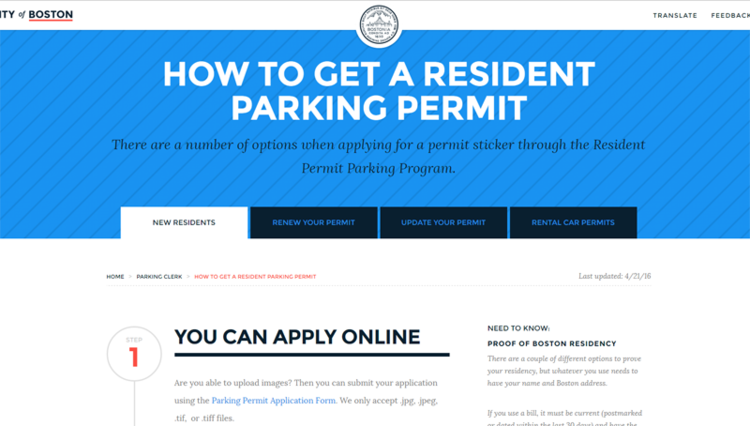This image is a detailed screenshot of the Boston Resident Parking Permit Program website, where residents can obtain parking permits. The page's design features a primarily white background with blue and black accents for emphasis.

At the top right corner, there are options to translate the page and provide feedback, enhancing usability and accessibility. The upper section of the page has a visually distinctive blue rectangle background adorned with diagonal gray lines running from the top right to the bottom left. This section prominently displays the title "How to get a resident parking permit" in clear white text.

Directly below this informative header, additional context is provided in blue text, stating, "There are a number of options when applying for a permit sticker through the resident permit parking program." 

Navigation buttons are situated underneath this text, allowing users to switch between different sections of the permit application process. The "New Residents" page is currently active, highlighted in white. Adjacent buttons, shaded in dark blue or black, guide users to pages for renewing permits, updating permits, or acquiring rental car permits.

The New Residents section features specific instructions, including steps to apply online, necessary information to know, and a requirement to provide proof of Boston residency. A convenient link facilitates the application process, ensuring users can easily proceed with their permit request.